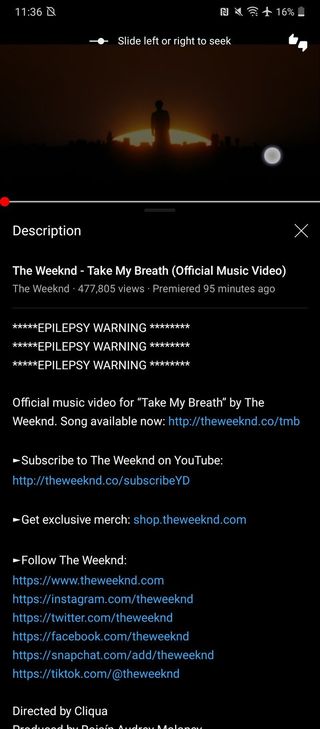The image is a screenshot of a cell phone displaying information about a video. The screen has a dark background with predominantly white text, creating a clear contrast. At the top, the time is displayed as "11:36." The image features a background scenery depicting a sunrise behind a silhouetted person and city skyline.

Centered on the screen is a red dot, indicating that the video is yet to be played. The text instructs users to "slide left or right to seek." The main content describes the video as "The Weeknd - Take My Breath (Official Music Video)," which premiered 95 minutes ago and has garnered 477,805 views. Following this, there is an "epilepsy warning" repeated three times vertically in capital white letters accompanied by star icons for emphasis.

A detailed description follows, mentioning that the official music video for "Take My Breath" by The Weeknd is now available. A hyperlink is provided: "http://theweeknd.co/tmb". Additionally, viewers are encouraged to subscribe to The Weeknd on YouTube, with another link provided, and to get exclusive merchandise through a separate hyperlink.

Subsequently, there are calls to follow The Weeknd on various social media platforms, including Instagram, Twitter, Facebook, Snapchat, and TikTok, each linked via a respective hyperlink. It is noted that the music video was directed by CLIQUA (spelled C-L-I-Q-U-A). The bottom part of the text is cut off, leaving some information missing.

Whether the screenshot is from YouTube is unclear, as there is no explicit mention of the platform within the captured text, only a suggestion to subscribe to The Weeknd on YouTube.